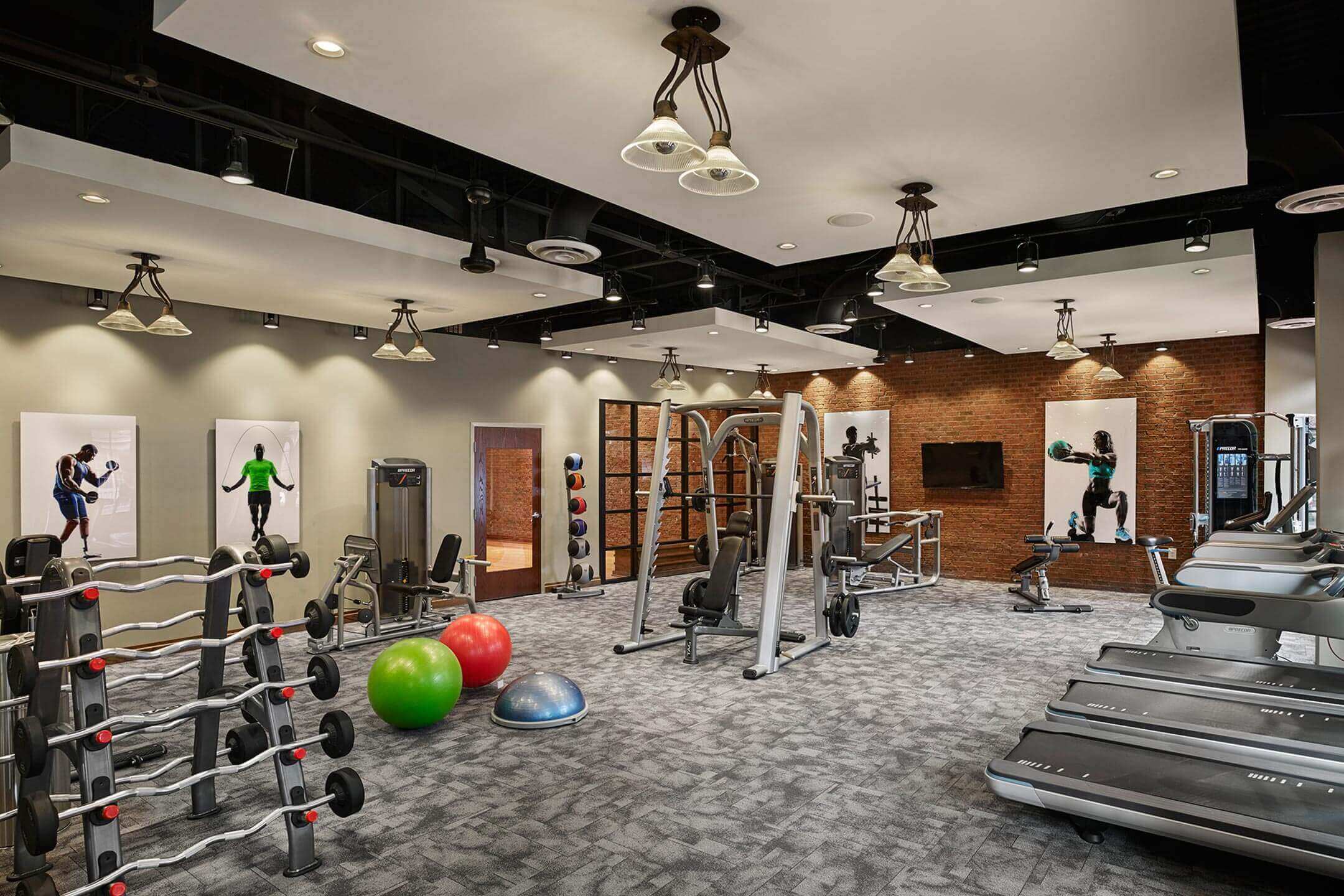The image depicts a well-equipped fitness area, likely from a small gym in a hotel or an apartment building. The gym features a variety of exercise equipment including treadmills, stationary bicycles, an elliptical machine, several weight training machines, and a selection of free weights such as dumbbells and barbells. Notably, there are also medicine balls and large stability balls of different colors scattered around. The room has a mix of painted and brick walls, with one brown painted wall and another made of exposed bricks adorned with athlete imagery. Additionally, one of the walls includes a TV screen, possibly for virtual workout sessions. The center of the gym features a machine with a chair for weight lifting or pulley exercises. To the left, there is a white wall with a brown door, flanked by a variety of workout equipment and additional imagery. The floor has a carpet with a floral design, enhancing the aesthetic appeal of this fully furnished gym space.